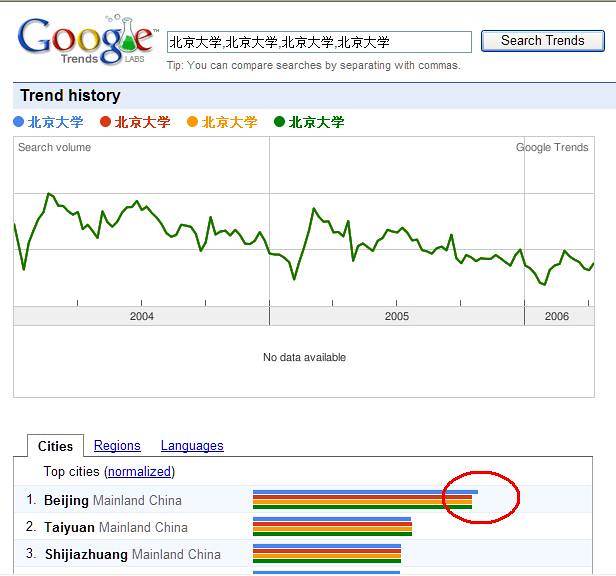This detailed image appears to be a screenshot of a Google Trends Labs interface, likely from a computer. In the top left corner, the Google logo is visible, accompanied by "Trends Labs." Nearby is a search bar containing Chinese text, next to a button labeled "Search Trends." Below the search bar, a tip is provided in English: "You can compare searches by separating with commas."

The main visual element is a "Trend History" line graph, with a blue, red, yellow, and green legend, each color-coded label written in Chinese. The graph displays data spanning the years 2004, 2005, and 2006, with a consistent green line traversing the years.

At the bottom of the graph, a tab section offers options like Cities, Regions, and Languages, with "Cities" currently selected. This tab lists "Beijing" as number one, followed by "Taiyuan" and "Zhejiang," each corresponding to a mini graph. The entire interface is predominantly in Chinese, with key functions and tips in English, suggesting a Chinese-oriented application for tracking and comparing regional search trends over time.